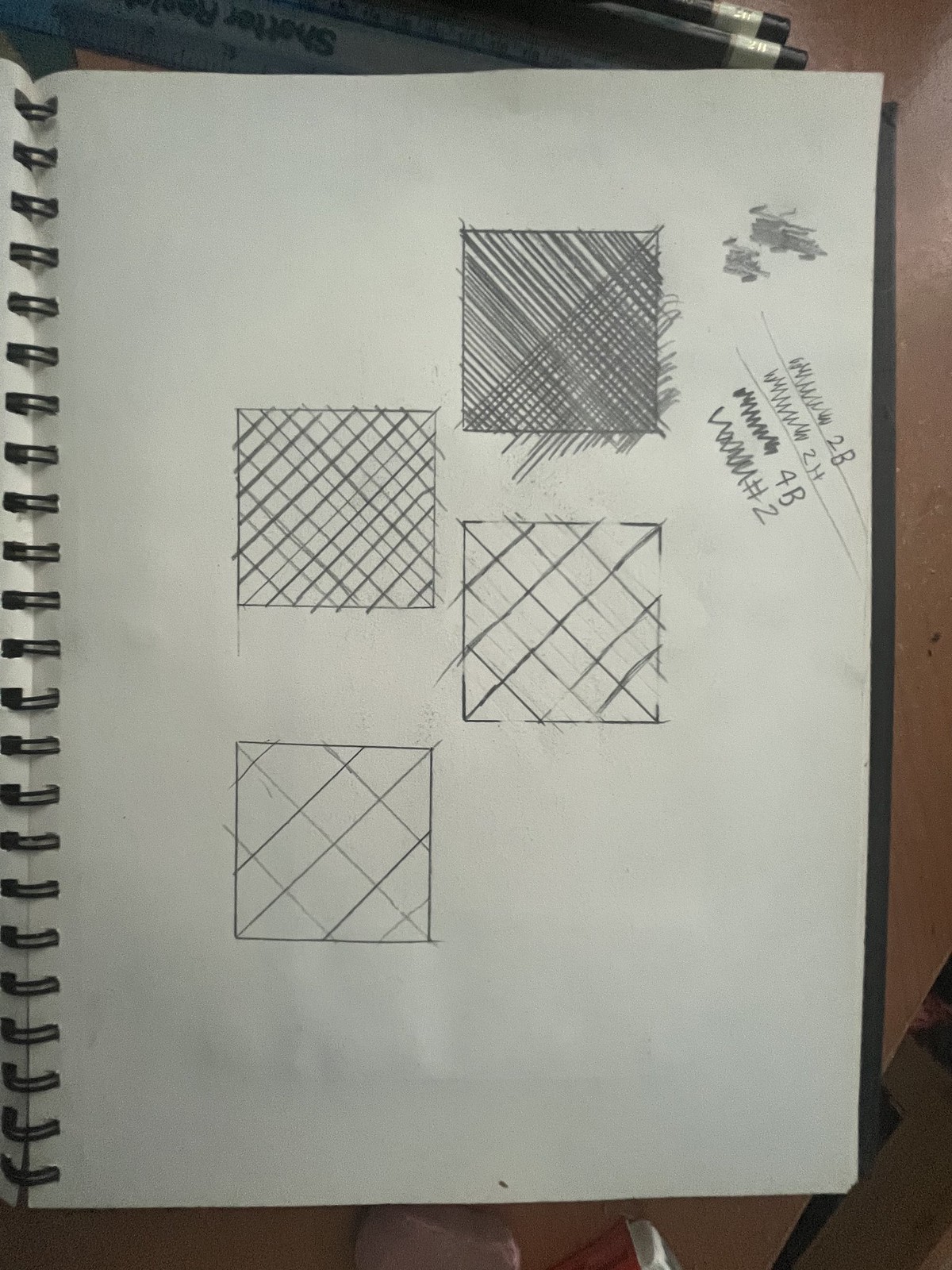A detailed close-up photograph depicting a black spiral-bound sketchbook, open to the right-hand page only. The spiral binding, also black, is clearly visible, as is the black cover of the sketchbook. The visible page features an array of cross-hatching exercises, organized into four distinct squares with varying densities of cross-hatching. The top right square displays dense and heavy cross-hatching, whereas the square directly below it has more widely spaced lines, creating a less intense effect. Further, the bottom right square adopts an even more spacious pattern, resembling a checkerboard due to the significant gaps between the lines. The bottom left square demonstrates the most open cross-hatching, with approximately ten visible diamonds formed by the intersecting lines. In the top right corner of the page, the artist has tested different pencil leads, ranging from 2B to 4B, showcasing variations in shading and texture.